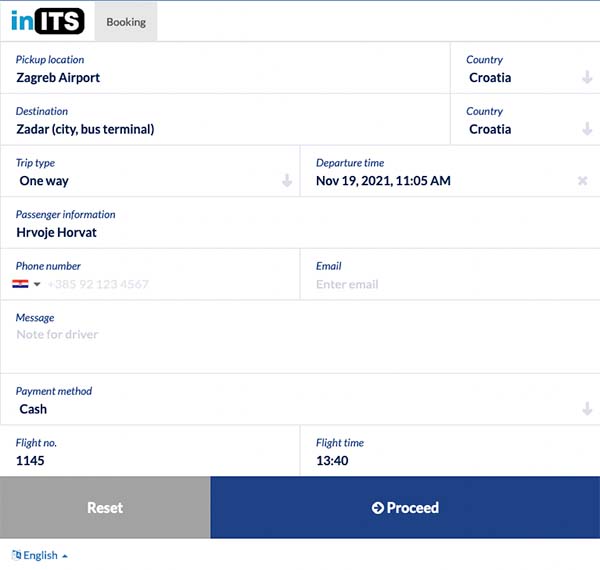A screenshot of a Croatian booking website is displayed, showing a detailed reservation form for a one-way trip. The form features a clean interface with a black-and-white background and white lettering, complemented by gray accents. 

The booking details are as follows:
- Pickup Location: Zagreb Airport, Croatia
- Destination: Zadar City Bus Terminal, Croatia
- Trip Type: One Way
- Departure Time: November 19th, 2021, at 11:05 AM

Passenger Information is provided:
- First Name: Hrvoje
- Last Name: Horvat
(No phone number or email is entered)

Other fields include:
- Note for Driver: [Blank]
- Payment Method: Cash
- Flight Number: 1145
- Flight Time: 13:40

At the bottom of the form, two buttons are present:
- Reset (in gray)
- Proceed (in blue, accompanied by an arrow)

Additionally, there is a translation button, which currently indicates the form is in English. This booking site clearly showcases an interface for scheduling travel between Zagreb and Zadar in Croatia, combining both bus and flight information.